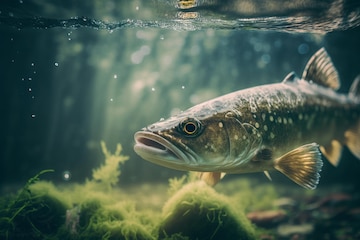The image depicts an underwater scene with a clear, crystal-blue hue. Dominating the middle to the right side of the photo is a catfish, colored in a mix of gold and black with white spots. The catfish is swimming leftward, its mouth slightly open, with its tail and fins trailing off the frame on the right. Surrounding the fish is a vibrant array of seaweed or green algae, particularly noticeable at the bottom of the image. There are also round areas of moss or possibly rocks covered in moss beneath the fish. In the distance to the left of the fish, a plant can be seen reaching upwards. At the top of the image, the water surface is visible, marked by a ripple that stretches from left to right. The clarity of the water reveals air bubbles dispersed throughout, contributing to the serene underwater ambiance. A brownish, oval-shaped object is noticeable in the top middle portion of the image, adding an element of intrigue to the scene.